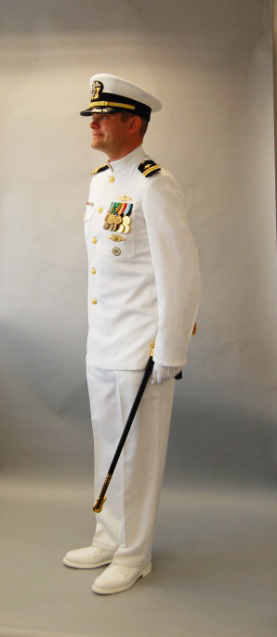The photograph depicts a Caucasian man standing in a room with a white or gray backdrop. He is dressed in an immaculate white military uniform, which includes a button-up shirt adorned with brass buttons, white pants, and white shoes. The man stands relaxed, facing to the left, and holds a black cane with gold markings in his left hand. His uniform features an array of medals on the upper left chest, along with epaulets on his shoulders and black cuffs. He is also wearing white gloves. He sports a white cap with a dark navy blue or black rim, topped with gold brocade and a central gold emblem, indicating his high rank. The man's friendly smile and relaxed stance suggest he is at ease while showcasing his distinguished military attire.